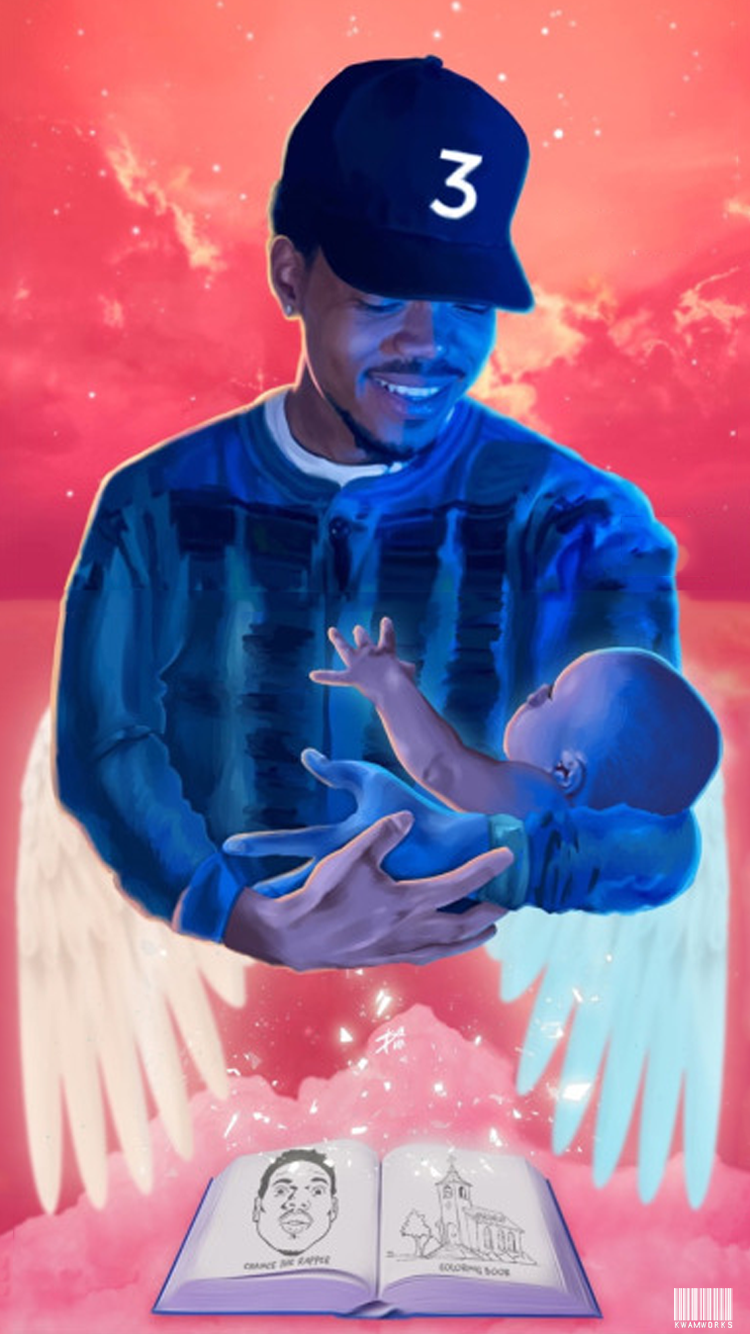This color image combines a photograph with computer-generated art, portraying a touching memorial scene. A black male, sporting a blue and black sweater with a white undershirt, and a navy blue baseball cap featuring the number 3, stands as the central figure. He has a mustache, beard, and an earring in his left ear. Cradled lovingly in his arms is a small baby, who reaches out towards him with its left hand. The man gazes down at the baby with a gentle smile. Emerging from his elbows are angelic wings that gracefully arc downwards, with bright white starlight-like sprinkles adorning the scene. Below them, a pink cloud mass holds an open book facing the viewer; the left page depicts a man's face, while the right illustrates a church building. The background transitions from a red to pink gradient sky, dotted with stars, enhancing the celestial and memorial essence of the image.